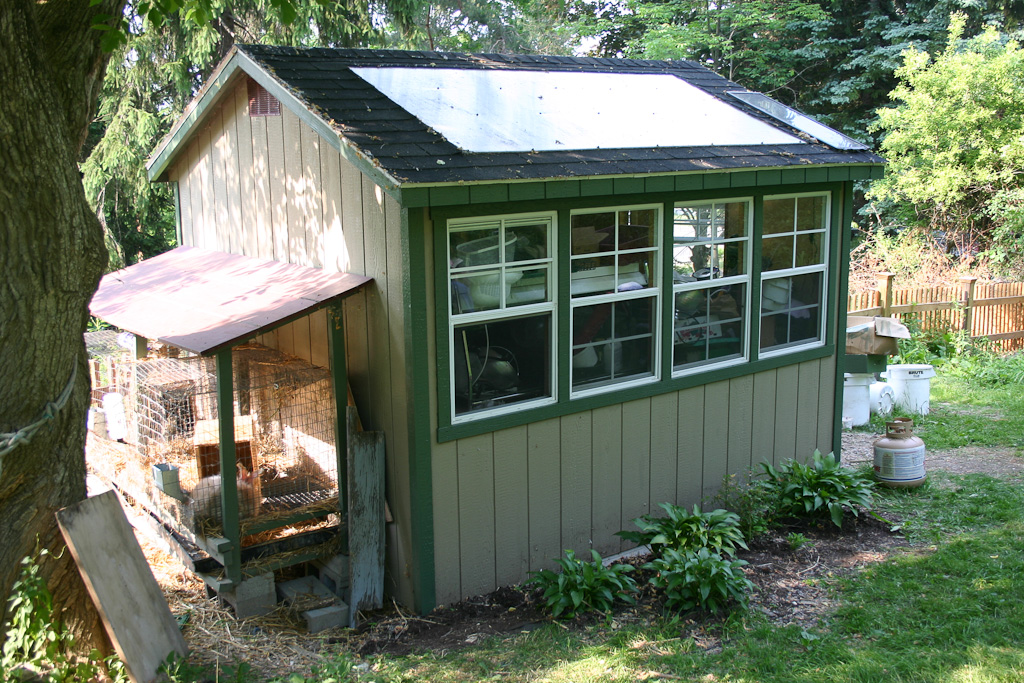This photograph showcases a cluttered outdoor shed situated in a rural backyard, encased by a wooden fence and surrounded by abundant trees. The shed, constructed of vertical planks of tan vinyl with green trim, features four windows—one of which is open—revealing a haphazardly stacked interior brimming with plastic containers and clothing. Mounted on its roof is a solar panel, and adjacent to the shed sits an empty propane tank, several white buckets, and a cardboard box. The base of the shed is bordered by green hosta plants, adding a touch of greenery to the scene.

On the left side, a wire-mesh rabbit coop with a red roof is affixed to the shed, housing a visible brown rabbit and several boxes. In front of the structure, patches of grass and shrubbery thrive under the shade of a large tree. A smaller tree to the left of the rabbit coop has a square piece of wood leaning against it. The overall setting is rural, indicated by the thick foliage in the background and the naturalistic elements surrounding the shed.